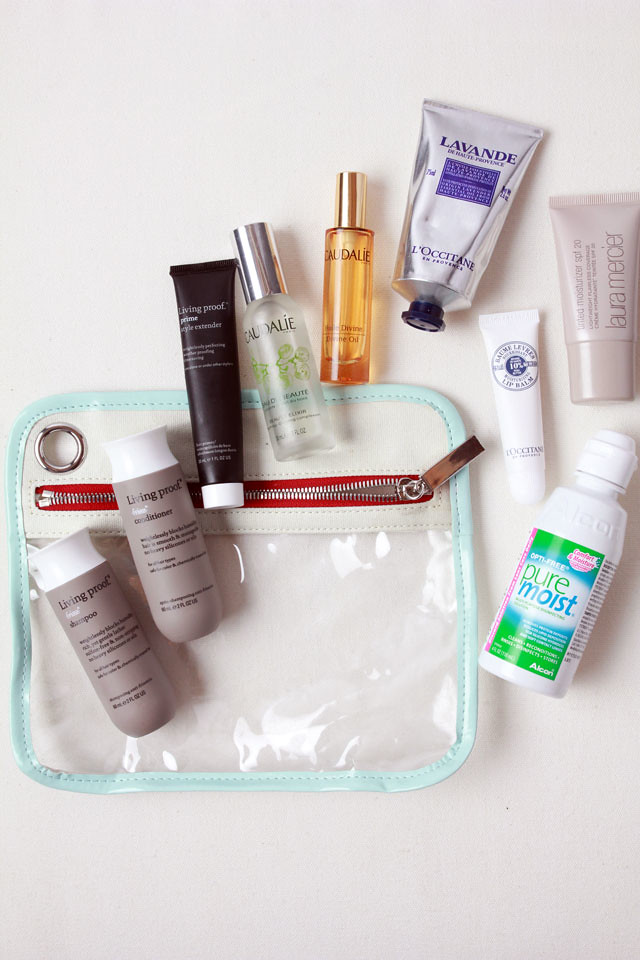The image showcases an assortment of personal care products meticulously arranged. On the left, there's a small 2-fluid-ounce bottle of Living Proof shampoo, characterized by its light brown packaging and white cap. Adjacent to it is another 2-fluid-ounce Living Proof product, this time a conditioner, mirroring the design of the shampoo. To the right of the conditioner lies a bottle of Living Proof styling product for hair. Further right, there is a serum bottle featuring a sleek silver cap. An orange bottle of hair oil stands next to the serum, adding a pop of color to the arrangement. A small bottle of Alcon Opti-Free Pure Moist Contact Lens Solution is also visible, providing eye care. Completing the line-up, a plastic bag with a convenient zipper is included, possibly for organizing the products.